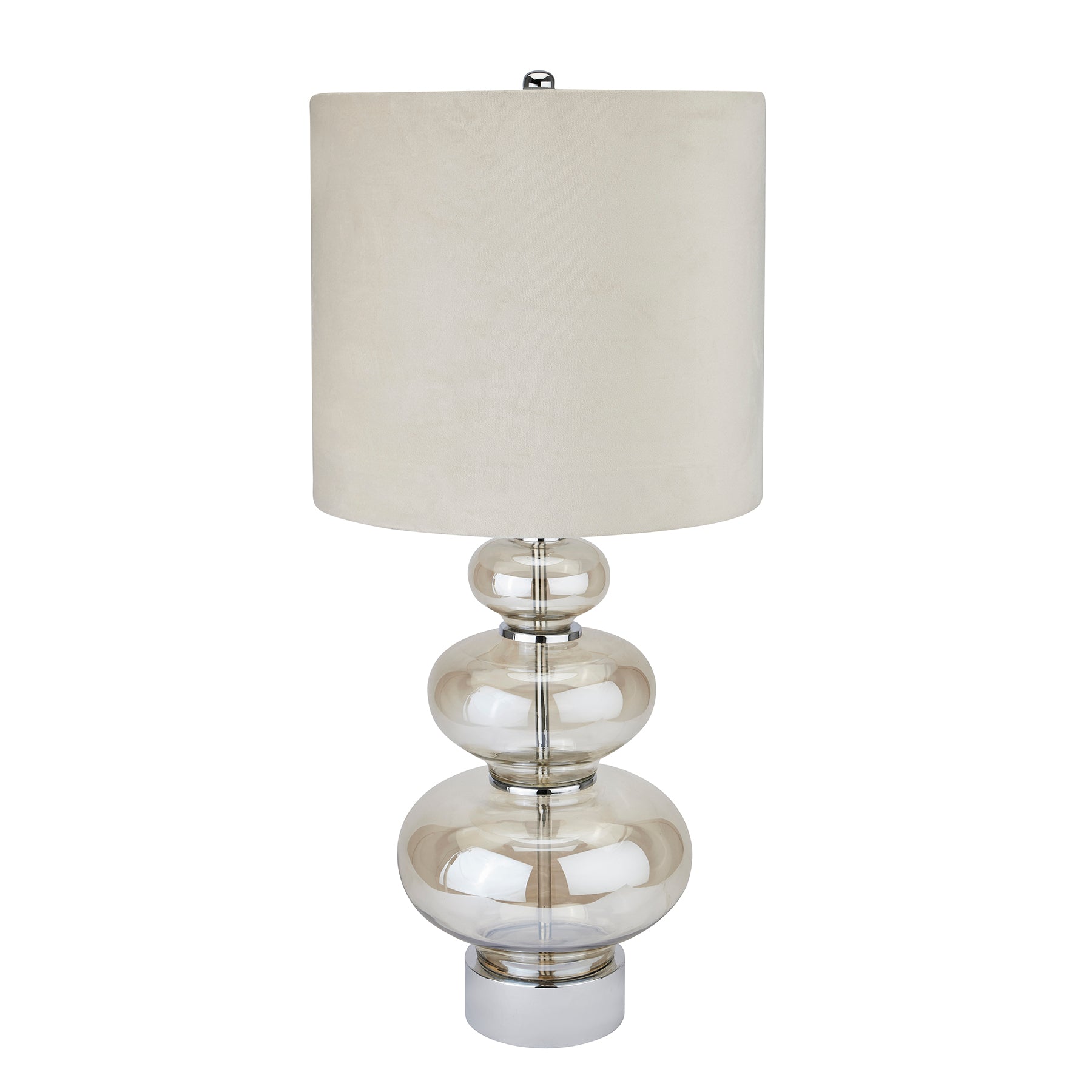This product photo showcases a creatively designed lamp, positioned centrally against a white background typical of a professional studio setting. The lamp features a white fabric cylindrical lampshade at the top, concealing a bulb. The unique base is composed of three reflective, glass-like spherical orbs, each progressively smaller as they ascend from the bottom. The largest orb sits at the base, with the smaller orbs stacked above it. The even, soft lighting enhances the reflective quality of the orbs, highlighting the intricate design. The colors in the image include various shades of white, darker white, brown, black, and gray. This setup draws attention to the lamp's distinctive and artistic style.